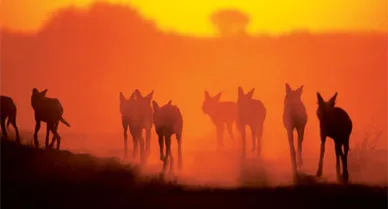In this striking, hazy photograph awash in red hues, the ground captures attention with its dusty surface, appearing almost black but speckled with tufts of grass. A pack of nine to ten wild animals, likely wolves, are distributed across the landscape, appearing to move in various directions. Some have lighter fur than others, adding depth to the scene. The backdrop features a distinctive tree line that transitions into a vivid, reddish-yellow sky, the result of a dramatic sunset. The sunlight’s glare bleeds onto the ground, enhancing the ambient, almost otherworldly glow. Far off on the horizon, faint silhouettes of trees or perhaps structures with mushroom-shaped tops add an intriguing element to the distant scenery. The overall atmosphere is one of serene wilderness bathed in an ethereal light.